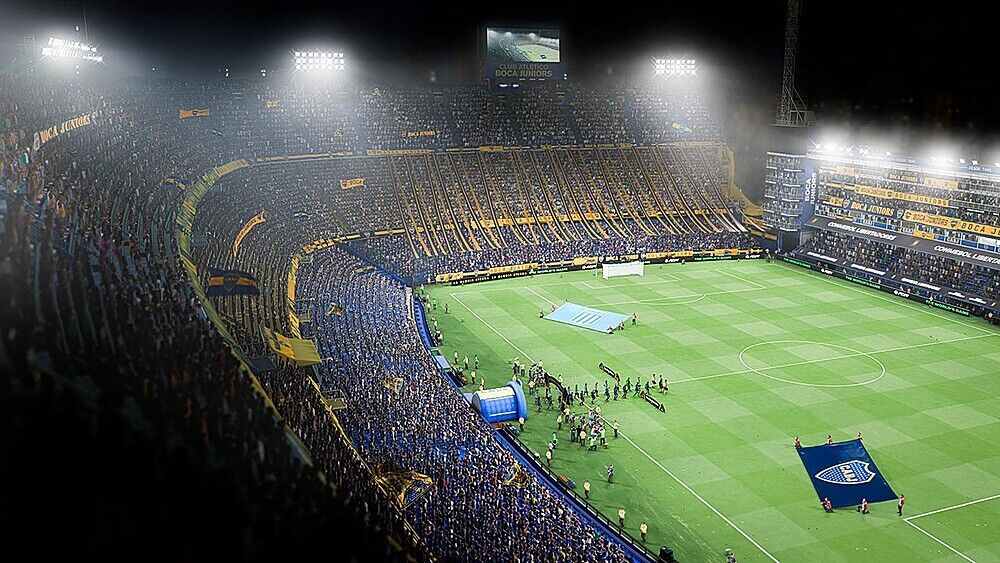This vibrant nighttime photograph captures the high-energy atmosphere of a soccer stadium bathed in artificial light. The expansive arena, adorned predominantly in blue and yellow, is filled with thousands of spectators eagerly awaiting the commencement of a match. On the lush green field, teams are emerging from a tunnel, setting the stage for an exciting event. In the bottom right-hand corner, six individuals hold a large flag displaying a shield with the letters "C-A-R-J" or "C-A-B-J," while in the bottom left-hand corner, another group of six carries a light blue flag with three indistinct stripes. The scene teems with anticipation as fans and players prepare for the opening ceremony, all underscored by the brilliant illumination from the stadium lights.